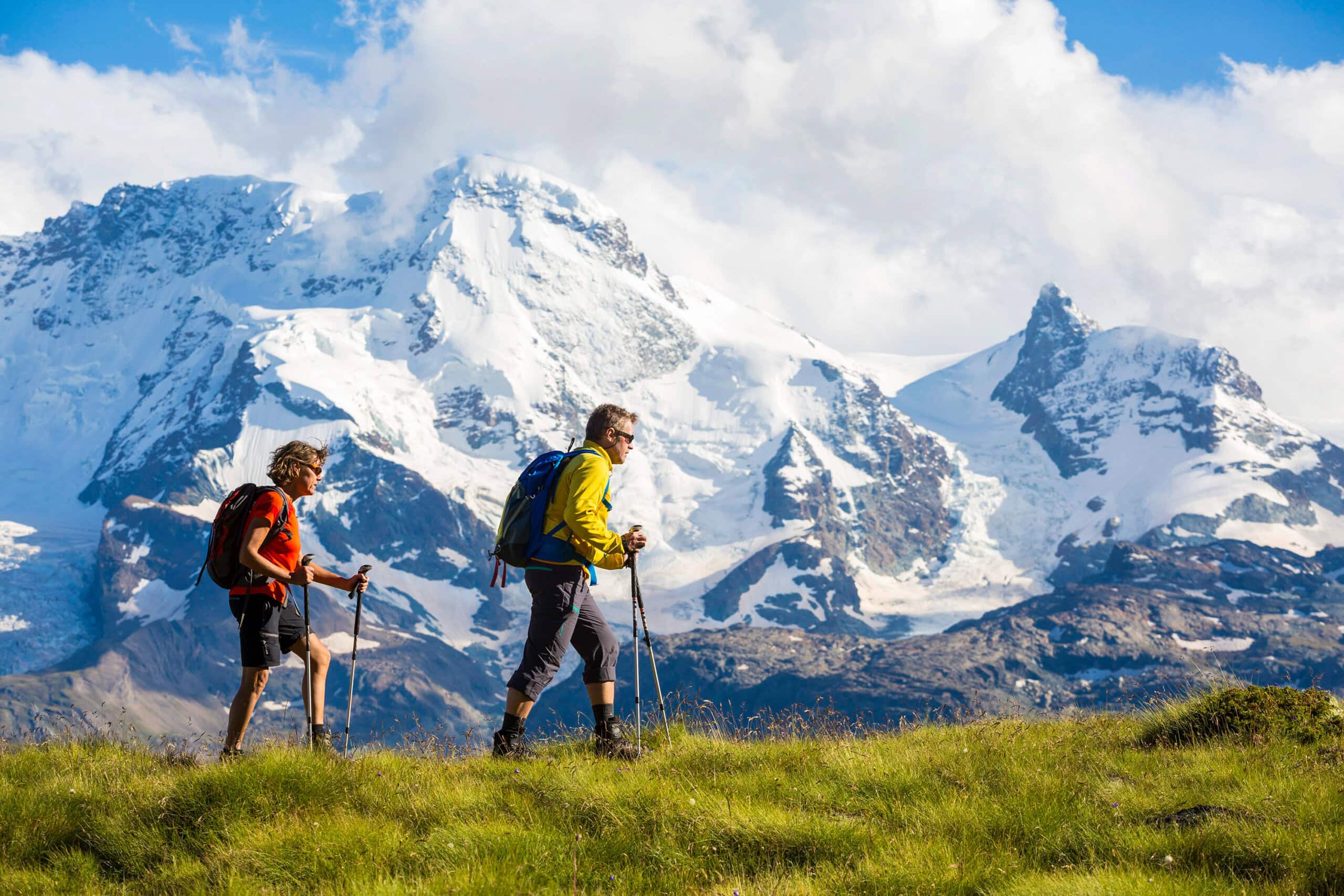The image captures a picturesque scene of a couple hiking up a grassy hill against a clear sky filled with soft, white clouds, imparting a romantic feel. Both hikers have short hair; the woman on the left is wearing a red t-shirt and black shorts, while the man on the right is dressed in a neon yellow jacket and black pants. They are walking from left to right within the frame. The background showcases majestic, snow-capped mountains bathed in sunlight, emphasizing the daytime setting. The lush green of the grass contrasts beautifully with the snow-covered peaks and the expansive, cloud-filled sky above.